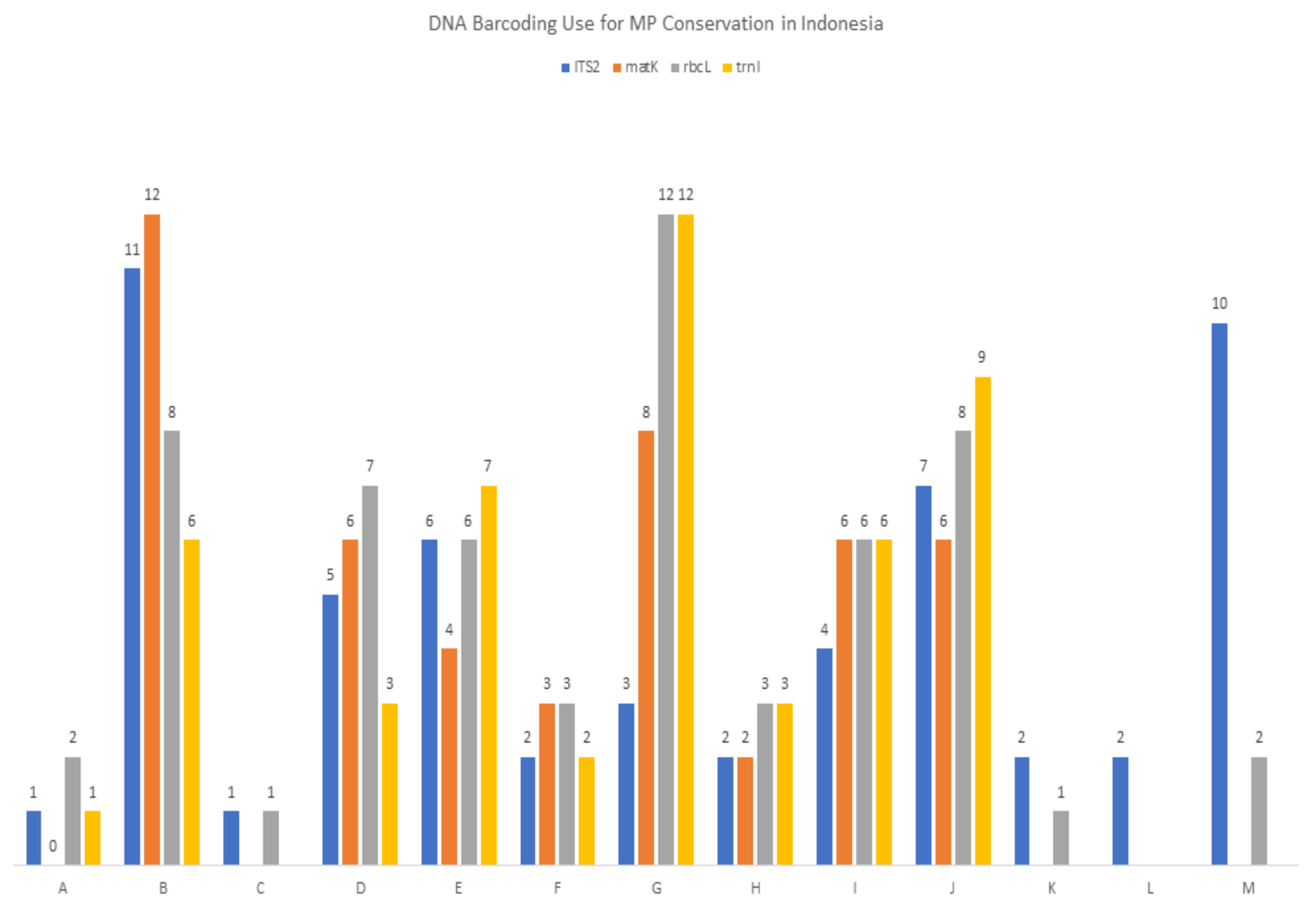This image depicts a detailed bar graph on a white background, which visualizes data related to the use of DNA barcoding for MP conservation in Indonesia. Across the top, in black text, the title reads, "DNA barcoding use for MP conservation in Indonesia." Beneath the title is a legend defining the color associations: blue for ITS2, orange for MATK, gray for RBCL, and yellow for TRNL. The graph itself features nine rectangular bars of varying heights in these colors.

The horizontal axis is labeled with letters from A to M, while the vertical axis is marked with numbers ranging from 0 to 12. The grid lines are light gray, and both the titles and axis labels are in blue. The bars represent different data points pertinent to the study, possibly illustrating levels of MP conservation success or related metrics across various categories denoted by the letters on the X-axis.